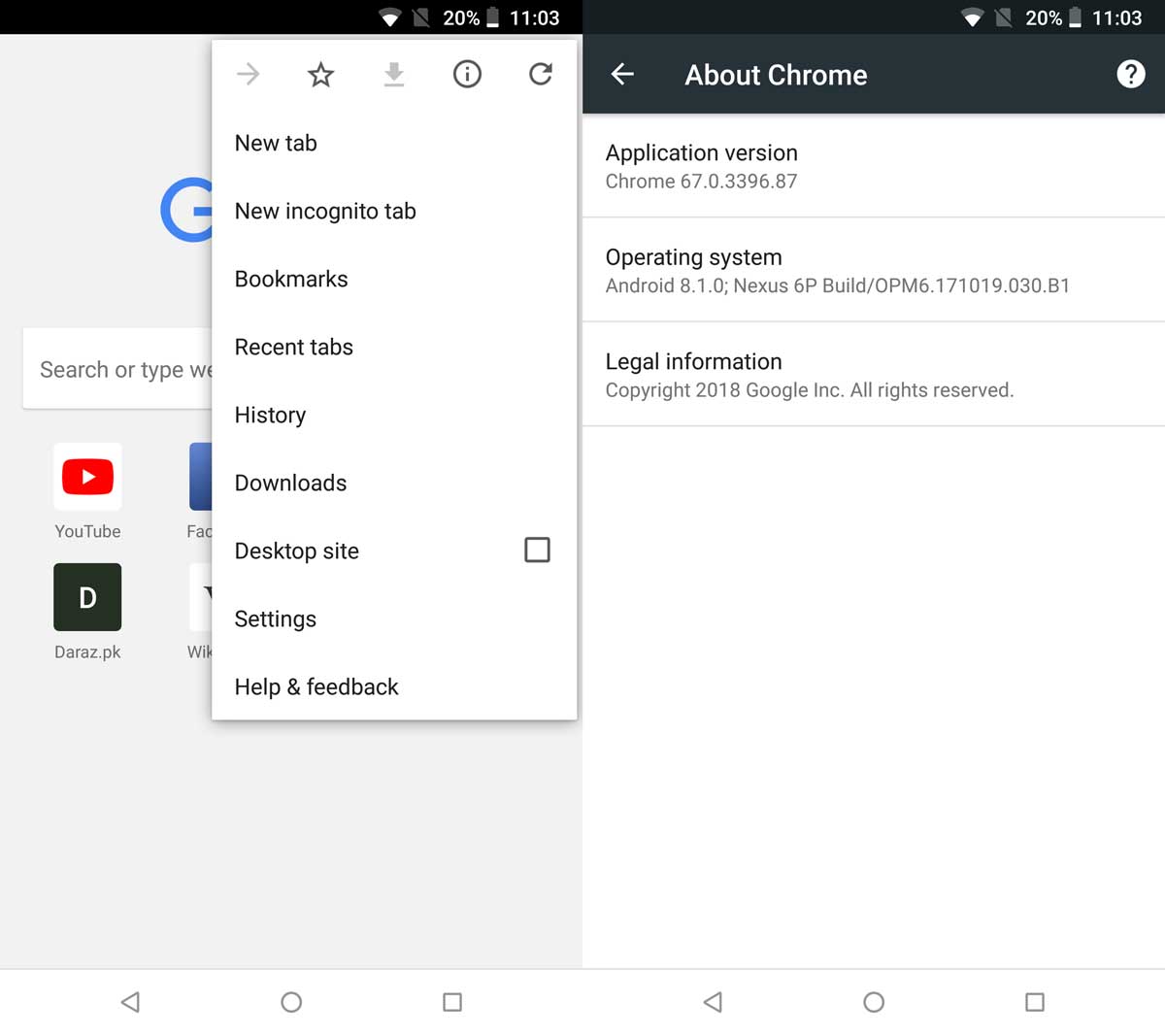This image contains dual side-by-side screenshots of a Nexus 6P device running Android 8.1.0. Both screenshots display a status bar at the top featuring multiple icons: a Wi-Fi icon, a "no SIM" icon, indicating there is no SIM card inserted, a battery level indicator showing 20% charge, and the time set to 11:03. 

In the first screenshot, a menu page is open, revealing an assortment of options. From top to bottom, these options include: 'Favourites', a 'Refresh' button, 'New Tab', 'New Incognito Tab', 'Bookmarks', 'Recent Tabs', 'History', 'Downloads', 'Desktop Site', and 'Settings'.

The second screenshot provides detailed information about the Chrome browser installed on the device. It lists the 'About Chrome' section and specifies the application version as Chrome 67.0.3396.87. The operating system is noted as Android 8.1.0, and the device is identified by its build number, Nexus 6P Build.